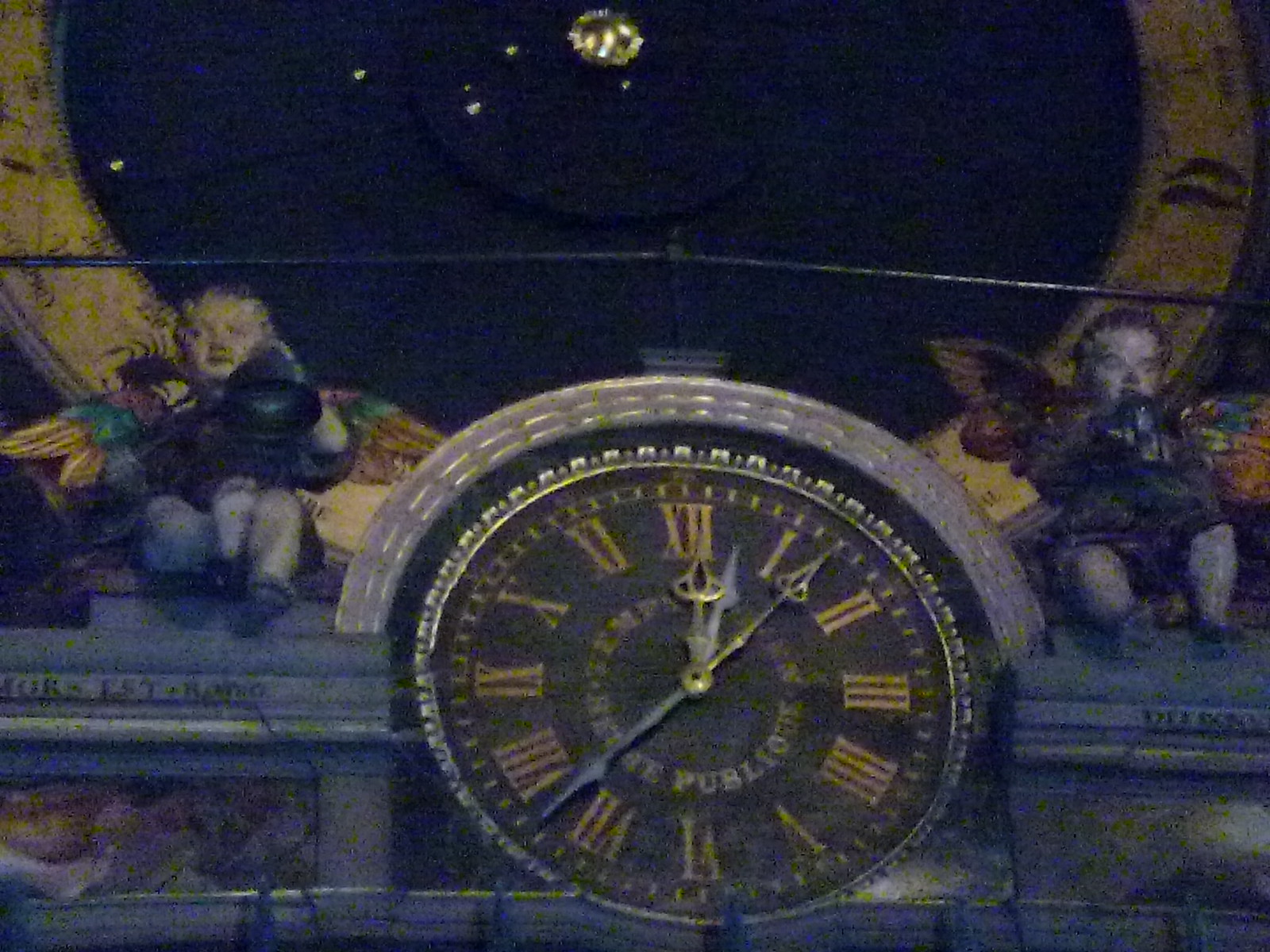The image captures a detailed view of a clock tower with an elaborate design. The centerpiece of the photo is a black clock face adorned with gold Roman numerals from 1 to 12. The clock features gold hands along with a silver, slender second hand. Encircling the clock face is a gray, rectangular background that appears aged. Written in a foreign language around the clock’s face are the words "TEMP, PUBLIS," among others. Above the clock, a silver metallic arch complements the design. 

Flanking the clock on both the left and right sides are small cherubic statues with wings, seated elegantly on ledges; these angelic figures add a touch of whimsy and classic artistry to the scene. The background further includes a large yellow circular shape featuring a black center and gold detailing, which is somewhat blurred but decorated with illustrations that seem to depict various objects, animals, and plants. The overall ambiance of the image is grainy and gray, hinting at its historical or artistic significance, potentially making it a part of a larger architectural piece or painting.